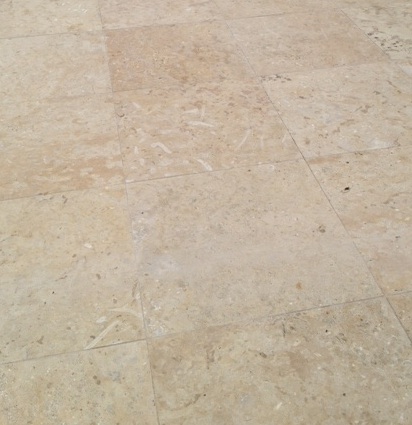The image showcases a simple, downward shot of a tiled floor, composed of large, rectangular marble tiles varying in color from light beige to medium light brown, with occasional white speckles and darker brown inclusions. The tiles display a natural, non-uniform pattern typical of aged or worn marble, suggesting a surface that has experienced considerable use, possibly akin to flooring found in modern train stations or upscale bathrooms. The grout or cement between the tiles is visible, securing them in place. The overall arrangement of the tiles and the intricate, unique designs on each one lend a natural and neutral aesthetic to the floor.